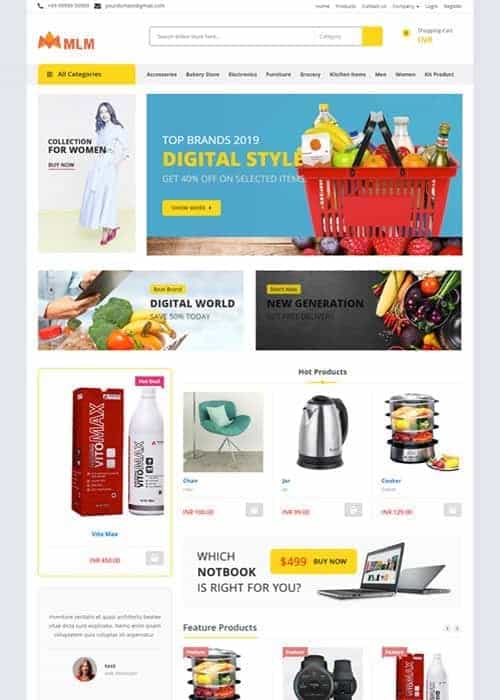The image appears to be a screenshot, likely from a tablet or desktop, displaying a website interface. The upper left corner includes an icon that looks like a telephone, though the accompanying phone number is unreadable. To its right, there is probably an email address, which is also unclear. Continuing to the right, there are six tabs; the last two tabs are legible and say "Sign In" and "Register."

The screenshot is bordered on the left and right by light gray vertical bars that stretch from top to bottom. The main content lies in the central section, which predominantly features a white background. Underneath the phone icon and email address is the company name, "MLM." To the right of MLM, there is a rectangular search bar with the words "Search" and a category drop-down menu labeled "Category."

Beneath the company name "MLM," a yellow rectangular background houses another dropdown labeled "All Categories." To the right of this dropdown, set against a light gray background, are several tabs. These tabs seem to be labeled "Accessories," "Bakery Store," "Electronics," "Furniture," and possibly "Brewery" or "Kitchen Home Meal."

Further down, below the "All Categories" dropdown, there is a section showing a collection for women with a call to action "Buy Now." Next to this section, there is an image of a red basket filled with grocery items like milk, olive oil, condiments, and various fruits. This section promotes "Top Brands 2019 Digital Style" in a yellow banner, with an additional callout, "Get 40% off on selected items."